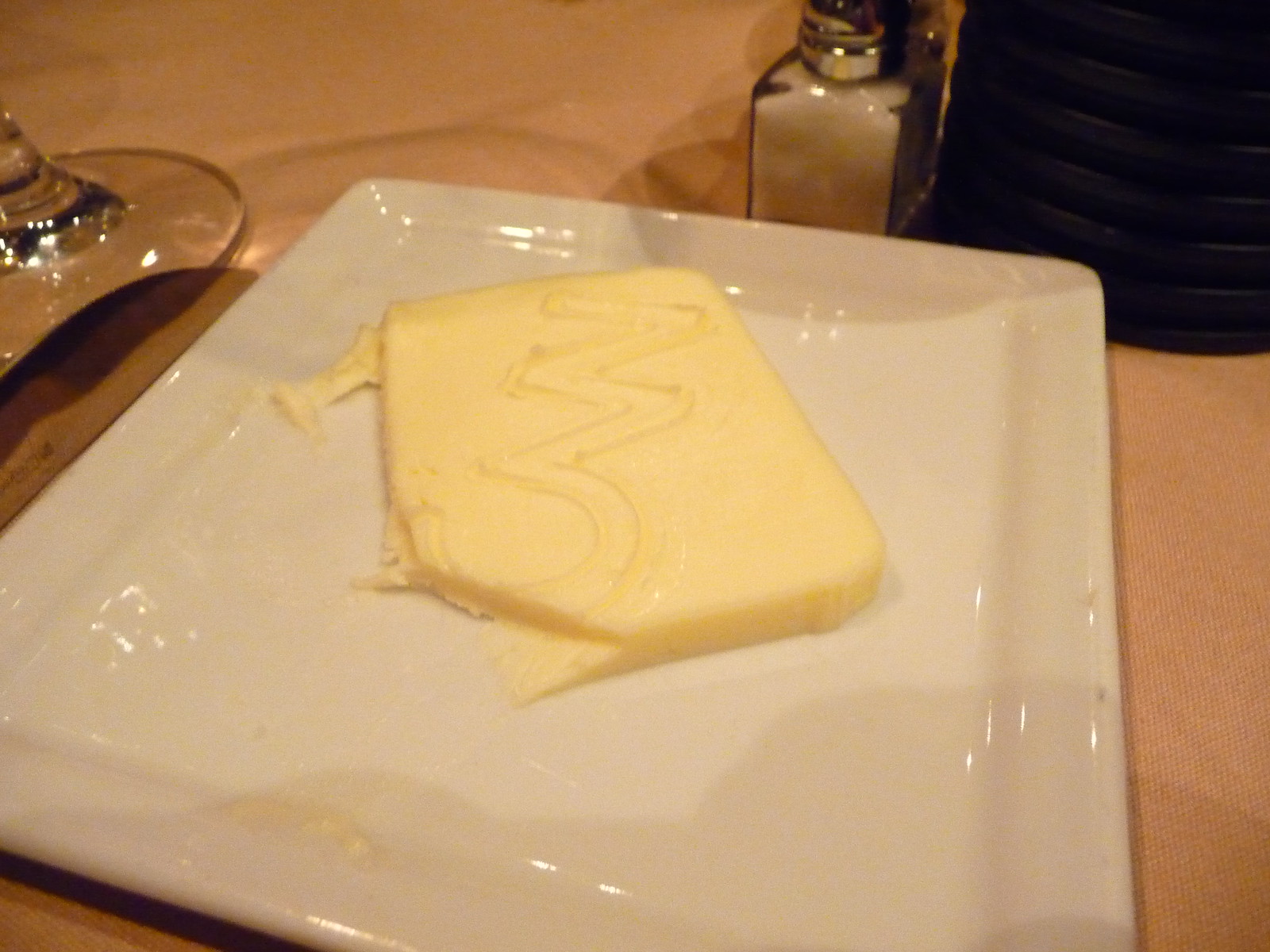The photograph captures a table setting with a peach or beige-colored tablecloth, possibly inside a dimly-lit restaurant. Dominating the center of the image is a white, ceramic square plate with raised edges. Positioned on this plate is a rectangular slab of butter featuring rounded corners and a distinct zigzag design that resembles a 'Z' connected to the top of a '3'. Part of the butter has been neatly cut away with a butter knife, leaving a straight edge. In the upper left corner of the frame, the base of a wine glass is visible. To the upper right, there is a small glass salt shaker filled with salt, alongside another indistinct shaker, likely containing pepper. Additionally, there is an unidentified black object or stack near the salt shakers. The photographer's shadow is cast on the bottom part of the plate, hinting at the low lighting within the shot.